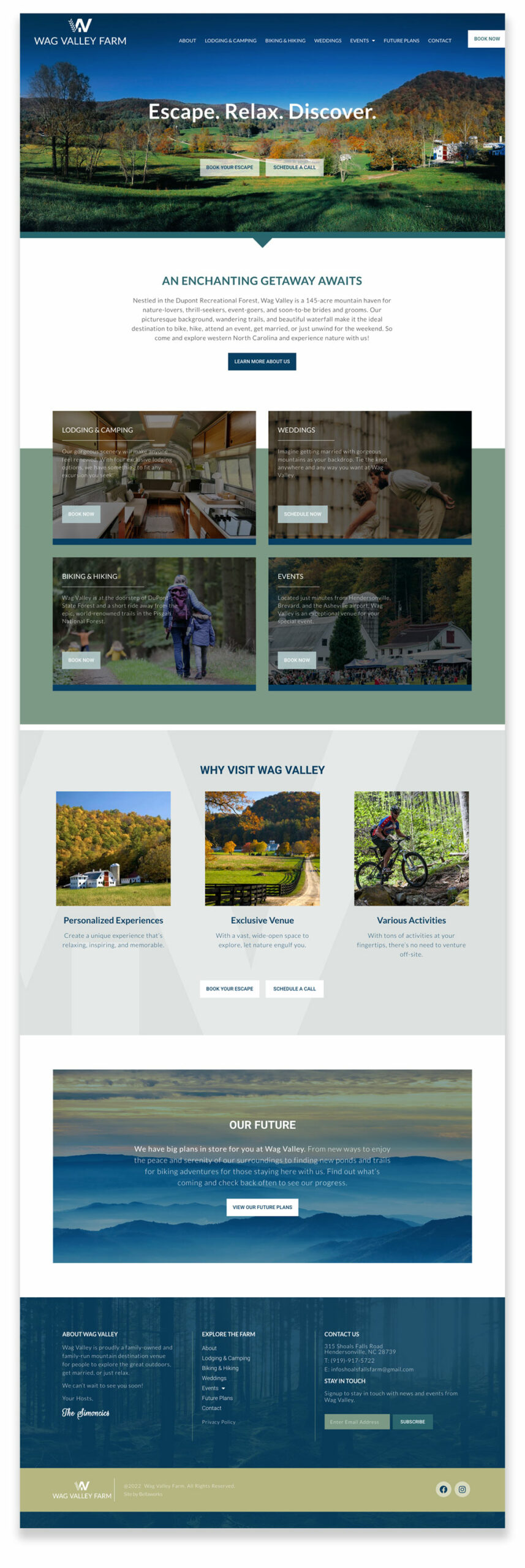The image is a screenshot of a vacation planning website, although the text is largely unreadable due to blurriness. At the top, there's a W-shaped icon, with the website title underneath it being indistinguishable. Accompanied by a scenic picture of a field with mountains and trees, the large white text across it boldly states, "Escape, Relax, and Discover." Below this image are two blurry white buttons and a similarly illegible white button in the top right corner.

Further down, a section titled "An Enchanted Getaway Awaits" is visible, followed by five lines of small, unreadable text and a blue button. Below this are four images arranged in a two-by-two grid showcasing different potential destinations: a venue lobby with an oval-shaped stage and seating, a couple sharing a kiss, an elderly person in gray attire possibly gardening, and a picturesque house with surrounding buildings, trees, a mountain, and either a lake or seashore.

Beneath this grid, the text "Visit Something Valley" introduces another set of visuals: a grassy field with a white farmhouse and trees against a blue sky, a fenced open field with a mountain backdrop, and a figure riding a mountain bike on a dirt path.

At the bottom of the screen, there are two large blue banners featuring a series of small, illegible words. The upper banner depicts bluish mountains fading into the horizon, and the lower banner contains additional unreadable text.